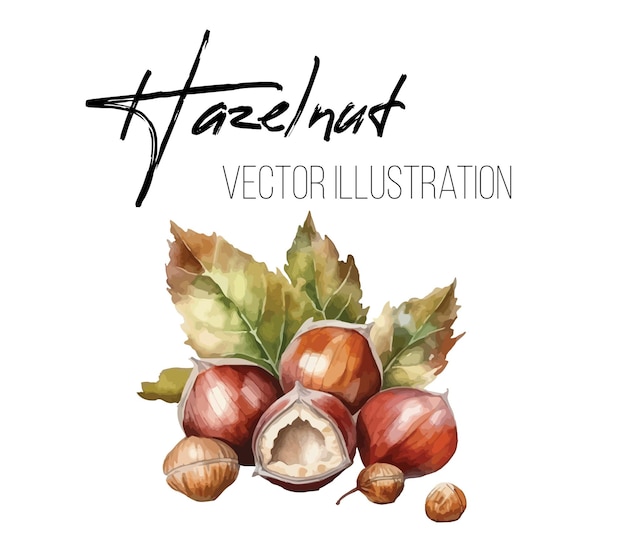This is a detailed digital illustration titled "Hazelnut," prominently displayed at the top of the artwork in a signature-style font. The image features a meticulously crafted depiction of hazelnuts, rendered on what appears to be a smart tablet. The focal points include four large hazelnuts, one of which is split open to reveal its white inner contents. Surrounding these are three smaller hazelnuts, positioned on their sides. The entire arrangement is set against a backdrop of green leaves, enhancing the natural aesthetic. The background is predominantly white, which highlights the vibrant, watercolor-like texture of the nuts and leaves. At the center, there is a sans serif watermark reading "Vector Illustration," indicating the digital nature of the artwork. The cohesive blend of artistic detail and modern digital techniques suggests this piece might be intended for use as a website graphic or logo.